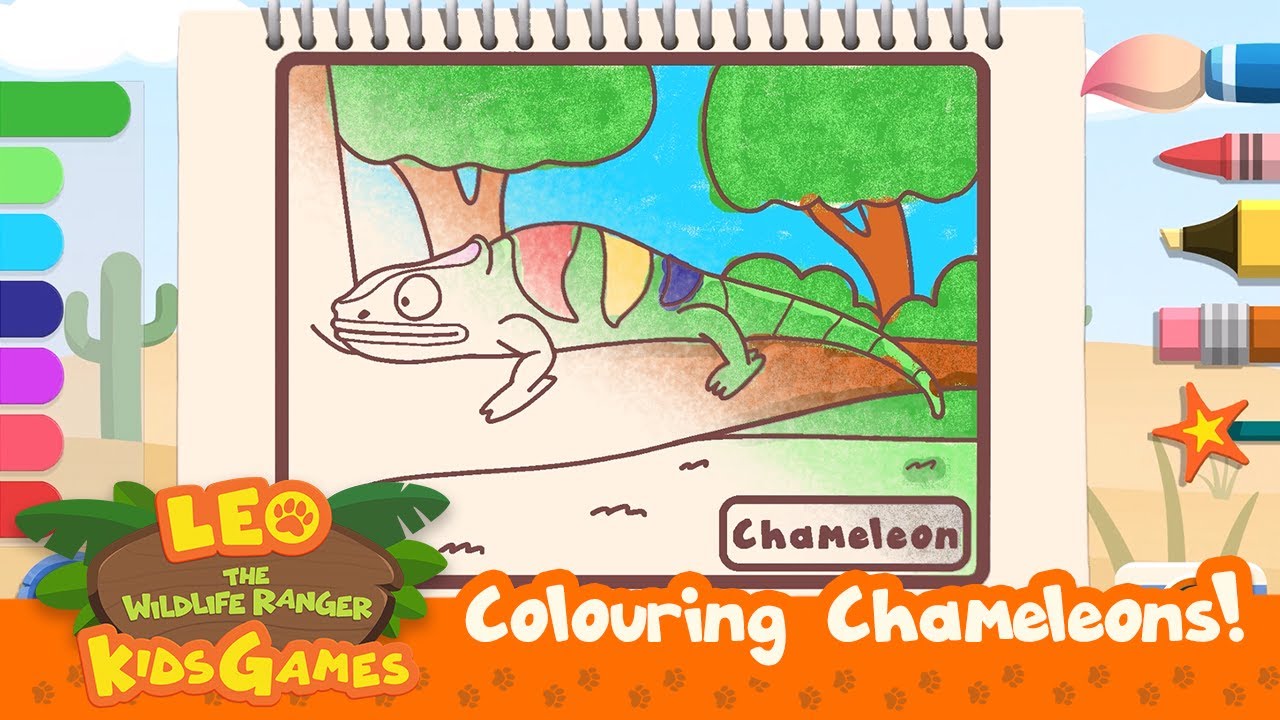The image displays the cover of a coloring book titled "Leo the Wildlife Ranger Kids Games: Coloring Chameleons," set against an orange banner with animal footprints at the bottom. Central to the image is a vibrantly illustrated chameleon perched on a brown branch, featuring a green body accented with red, yellow, and blue stripes. The chameleon's tail is segmented, and its white head is marked with pink at the crest. Surrounding the chameleon, you can see green-leaved trees with brown trunks and branches, a brown ground with patches of grass, and a distant sky. To the left of the image, a cactus and a series of color strips—green, blue, purple, and red—are visible. On the right side, various coloring tools, including a pink paintbrush, a red crayon, a yellow marker, a pencil with an eraser, and a magic wand with a star, are neatly arranged. The text "Chameleon" is boldly written in the bottom right corner, suggesting the final, uncolored touches to the drawing.